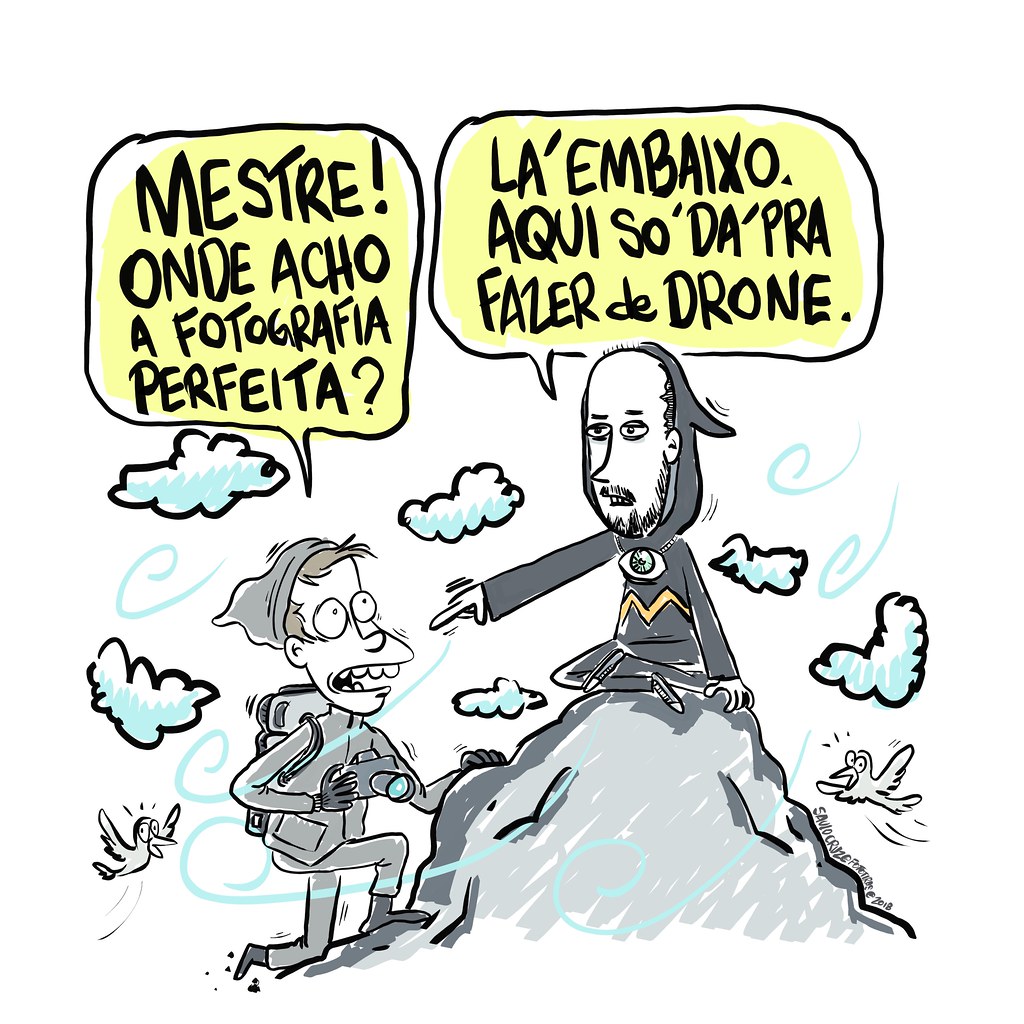This is a detailed colored cartoon or comic set against a white background adorned with white clouds accentuated by blue squiggly lines and swoopy blue lines denoting wind. Two birds hover with shocked expressions, seemingly amazed at the heights reached. At the peak of a lofty mountain, a hiker clad in a beanie, backpack, and gloves, with a camera around his neck, has finally completed his climb. He stands face-to-face with a wise man, who has a long beard and is dressed in a hooded robe adorned with an all-seeing eye medallion. The wise man, who is bald, sits cross-legged atop the mountain, extending his right arm toward the hiker. A yellow thought bubble contains black text in a foreign language, reading "Mistre Onde Acho a Fotografia Perfeita," The wise man responds with "Lá Embaixo Aqui Sou Dá Pra Fazer De Drone." The scene captures the essence of an enlightened encounter amidst the lofty, wind-swept heights.